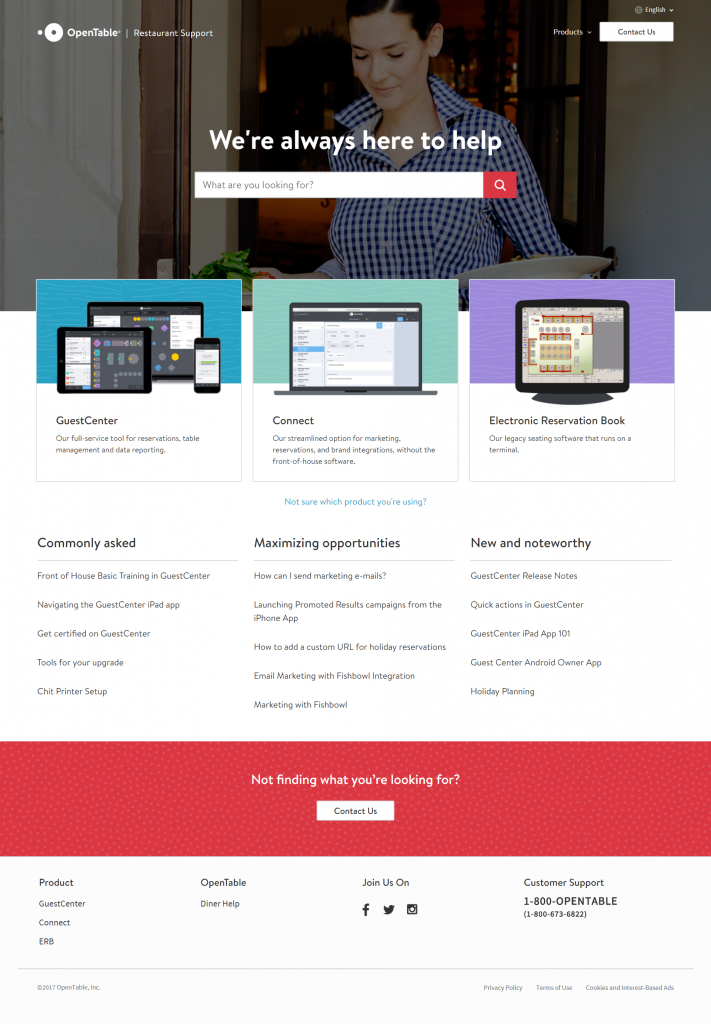The image appears to be a color screenshot taken from the OpenTable website. In the top left corner, the OpenTable logo is prominently displayed in white, with the accompanying text "OpenTable" also in white. On the right-hand side of the header, there's text that reads "Feature" next to a pull-down menu.

Dominating the central portion of the image is a picture of a woman with her eyes closed, looking downward. She appears to be exiting from her front door, about to step outside. She is dressed in a blue and white plaid button-down shirt. Overlaid on this image is the reassuring message, "We're always here to help."

Beneath this central image, there is a search bar with the prompt, "What are you looking for?" Below the search bar, there are three clickable options arranged horizontally: "Guest Center," "Connect," and "Electronic Reservation Book."

Further down, informational sections are presented in three columns. The first column, titled "Commonly Asked Questions," provides links to frequently asked questions. The middle column, labeled "Maximizing Opportunities," includes topics such as "How can I send marketing email?" The third column, "New and Noteworthy," features the latest updates and additions.

At the bottom of the image, there's a prominent red banner with the message, "Not Finding What You're Looking For? Contact us," encouraging users to seek further assistance if needed.